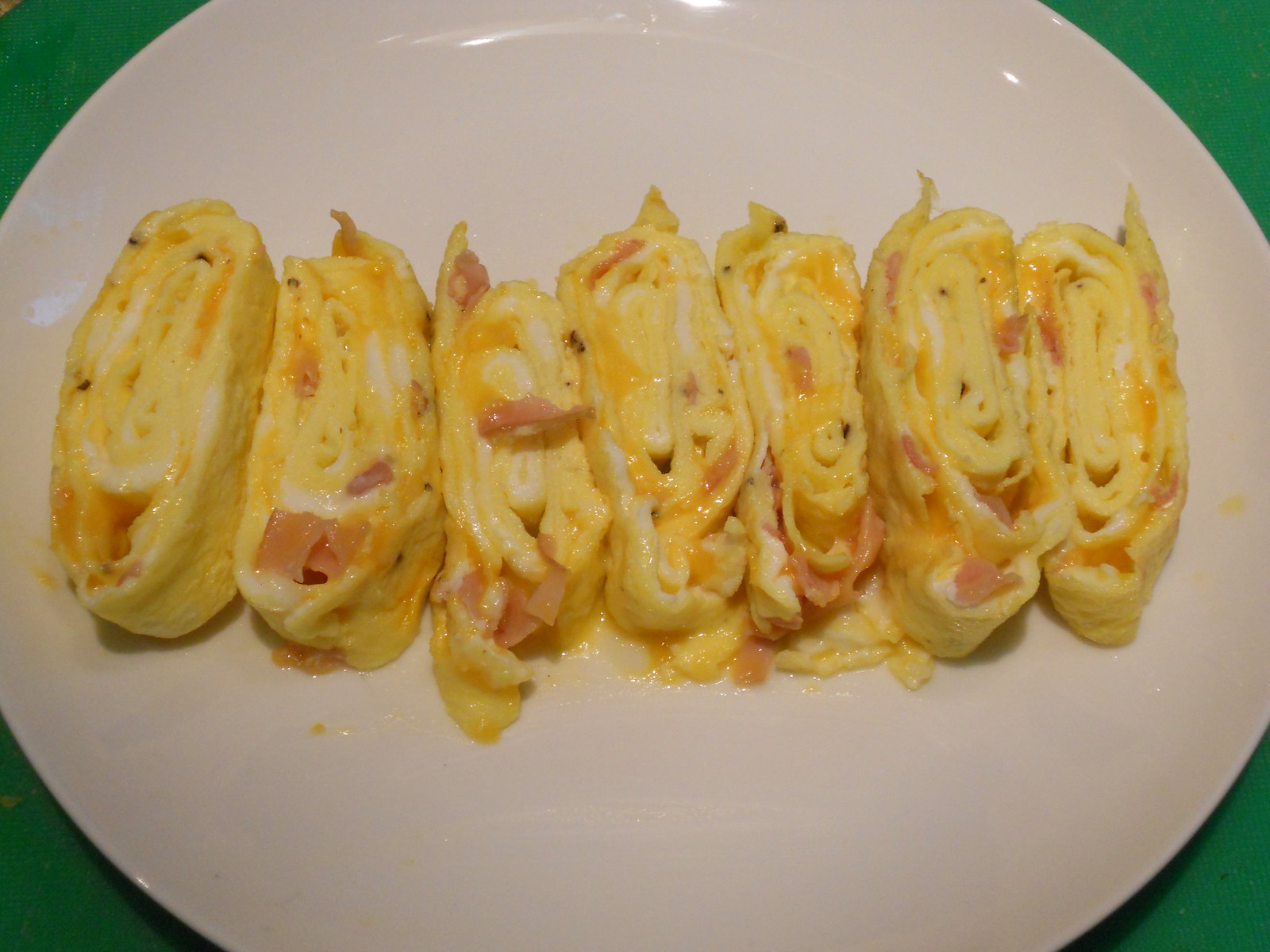The image features a freshly prepared breakfast platter centered around a large egg omelette sliced into seven smaller segments. Each piece of the omelette is stood on its side, revealing a detailed cross-section of its contents. The omelette has been stuffed with chunks of ham, white cheese, and yellow cheddar cheese, giving a layered, spiral appearance. The pieces are meticulously arranged side by side, running horizontally from left to right on a pristine white serving plate. The background appears to be a green tablecloth, adding a contrast to the bright egg dish. Notably, there's a reflection on the plate and eggs, likely from a camera flash, and a few scattered specks of egg hint at the dish's homemade nature.